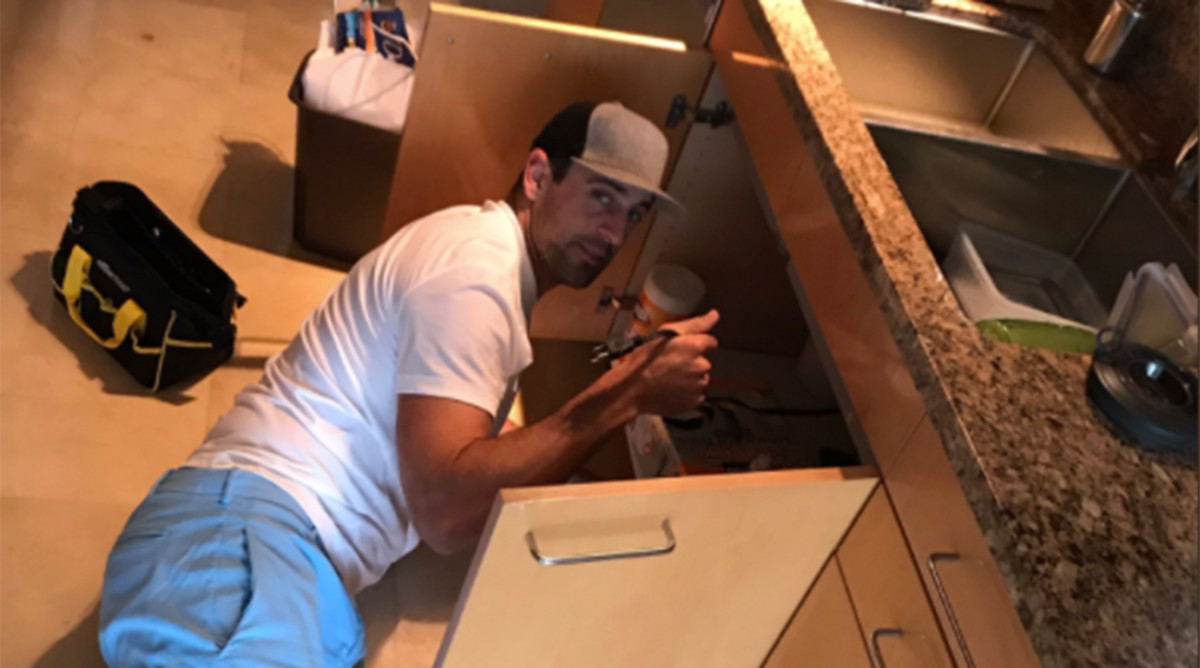In the photograph, a person is fixing a sink situated on a marble countertop on the right side of the image. The photo is slightly tilted, offering a dynamic perspective. The marble countertop features a double-basin sink made of a silver-gray material. The individual, who appears to be a white man with a goatee, is lying on his left side on the floor. He is dressed in light blue pants, a plain white T-shirt, and a gray and black baseball cap.

The man's proximity to the sink allows us to see the cabinet doors beneath the sink, which are open. These wooden doors have silver handles and reveal the under-sink area where the man is working. To his left, there is a black and yellow tool bag, suggesting that he is in the midst of repairs. The room's floor is tiled, adding to the clean, organized ambiance.

Additionally, a black trash can with a white liner is visible near the top of the image. Inside the sink are a couple of plates, one white and green and the other light green. The photo also captures part of the kitchen or bathroom cabinetry, which features brown drawers and cupboards that complement the marble countertop. The entire scene is well-lit, highlighting various elements that suggest a typical home repair scenario.